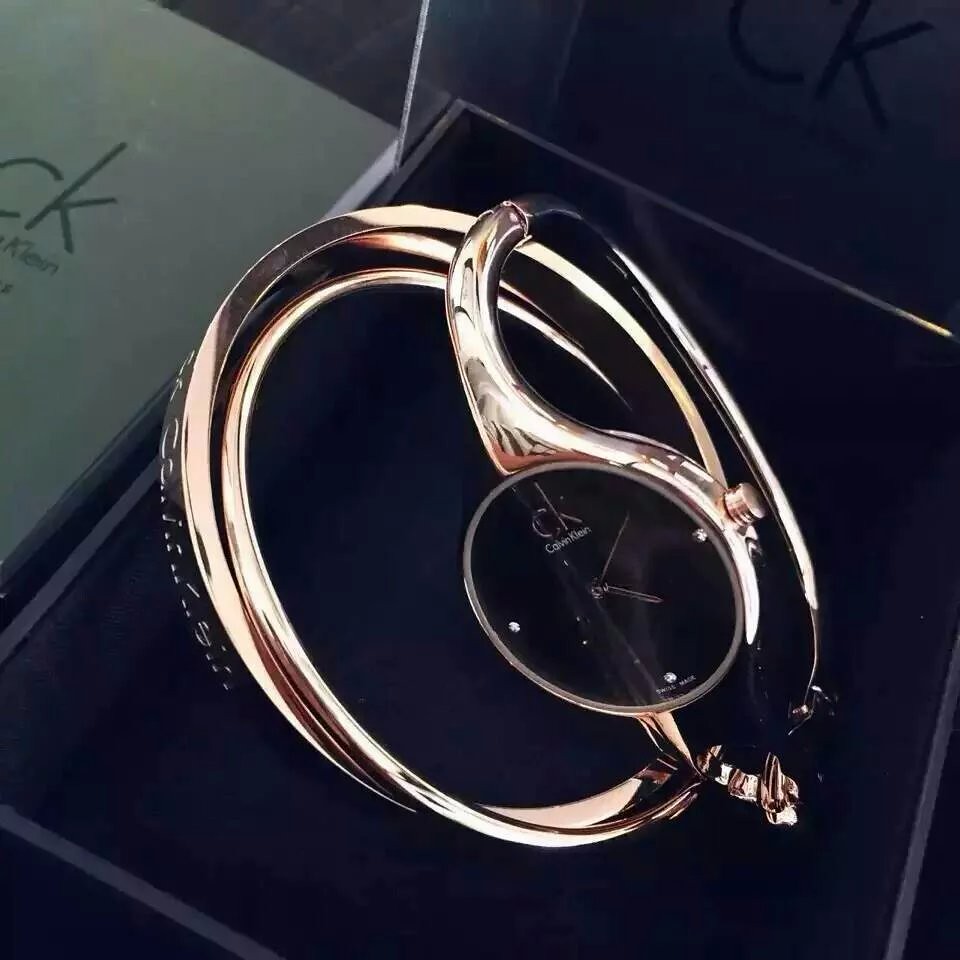The photograph portrays a close-up of a highly stylized Calvin Klein watch showcased in what appears to be a store display case. The watch, resting on a dark black velvet surface, is crafted from elegant rose gold metal and features a unique multi-band strap design, diverging from traditional single-strap watches. The case, which slightly tapers at the corners, stretches backwards on a diagonal angle towards the right. The black watch face is adorned with mini diamond-like stones elegantly positioned at the three, six, and nine o'clock markers, adding a touch of sophistication. The Calvin Klein logo is prominently displayed just below the CK insignia at the twelve o'clock position. In the background, the open back of the case fades out of the image, while the left side reveals another Calvin Klein logo on the surface of what looks like another box, enhancing the impression that these luxury timepieces are being meticulously displayed in a retail setting. The face of the watch is oriented towards the viewer, slightly tilted to favor the bottom left diagonal, inviting closer inspection of its refined details.